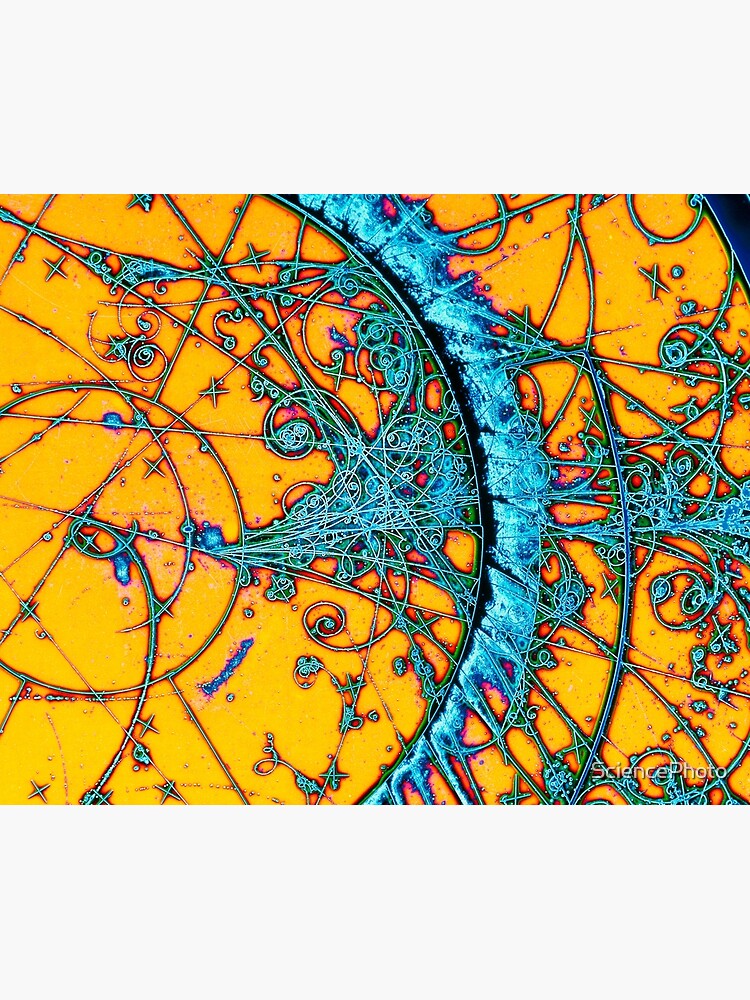The image depicts a striking and colorful close-up reminiscent of stained glass, featuring predominantly bright yellow and neon (turquoise) blue hues. The design is intricate, with various patterns and shapes, including numerous lines and curves. At the center lies a prominent crescent-shaped curve, which evokes the appearance of a half-sun. The black crescent is bordered by thicker blue lines at its base, and white lines outlined in blue that radiate outwards in different directions. The background primarily showcases a light orange color, with a small portion at the top right corner revealing a blue stripe and a black area. Despite the details, the overall image remains abstract and zoomed-in, making it difficult to identify its exact nature, although a note in the bottom right corner suggests it is a scientific photo.